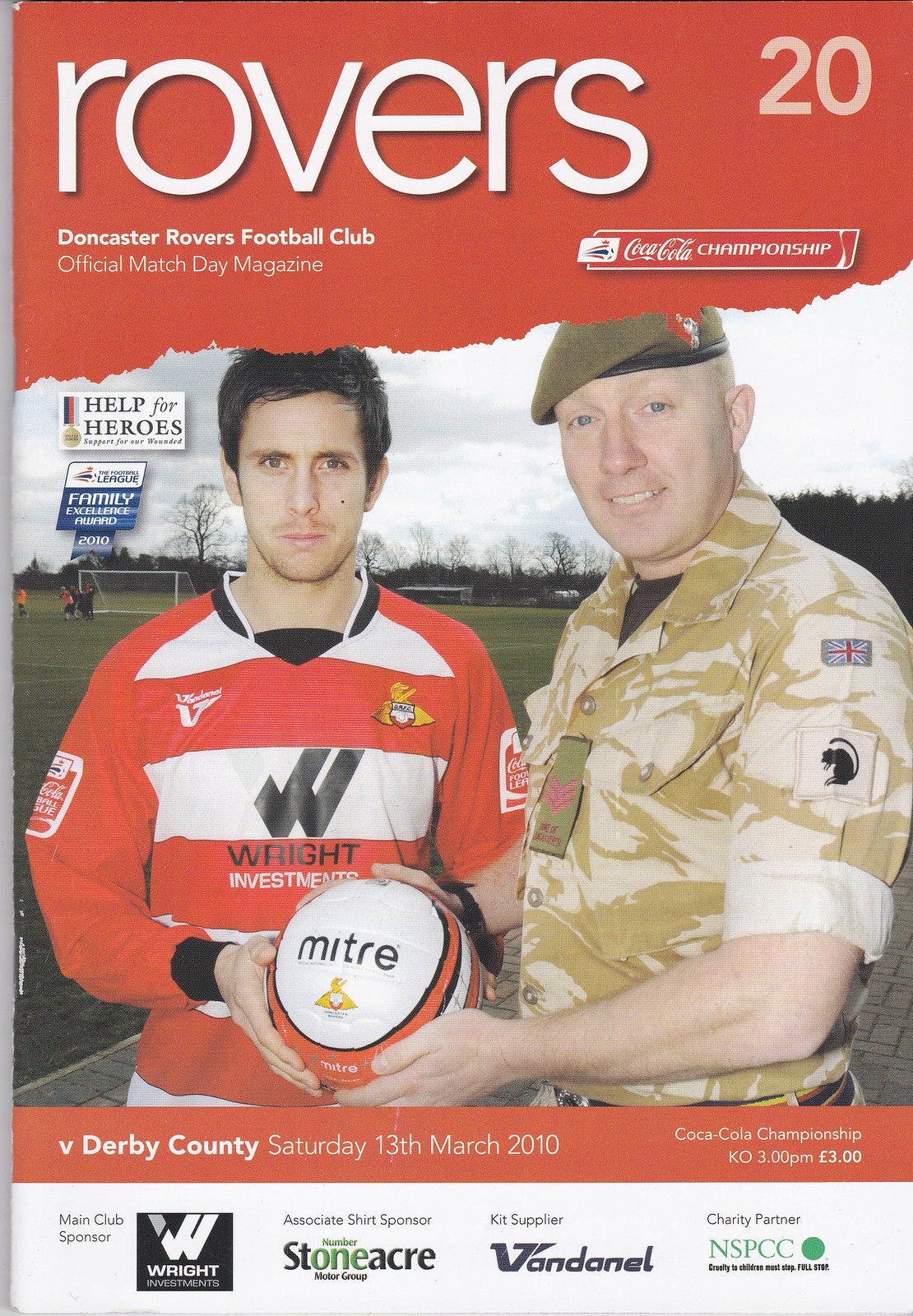This is a detailed, color image of the cover of the Doncaster Rovers Football Club official match day magazine for their match against Derby County on Saturday, March 13th, 2010. The primarily red and white cover is headlined with "Rovers" in bold white letters at the top, accompanied by the number 20 and the title, "Doncaster Rovers Football Club Official Match Day Magazine." Notably, the cover features a prominent photograph of two men. On the left is a soccer player donning a red and white jersey emblazoned with "Wright Investments," holding a soccer ball. Beside him stands a man dressed in a military camouflage uniform, also touching the ball, presumably representing the British Royal Army. To the left, there is a supporting message for "Help for Heroes," accompanied by an image of a medal, emphasizing support for the wounded. Below the photograph, the details of the match are highlighted with "V. Derby County, Saturday, 13th March 2010, K.O. 3 p.m., 3 pounds." The bottom section of the cover lists sponsors including Wright Investments, Stoneacre Motor Group (cleverly designed with the letters "O" and "N" forming the number one), Vandanale, and the NSPCC.